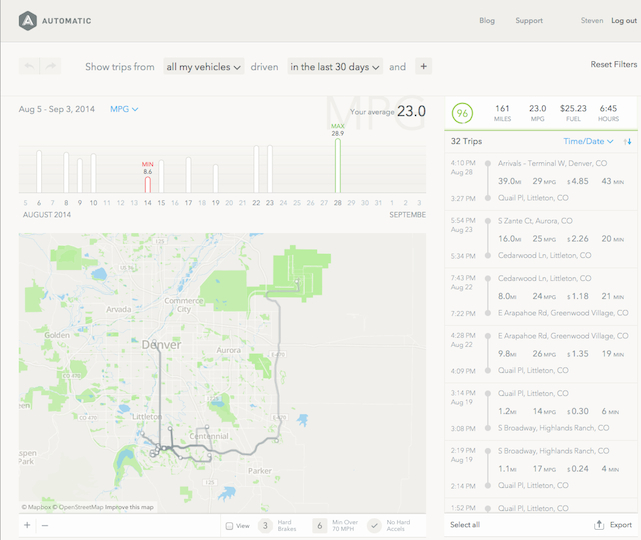The screen displays a detailed interface for monitoring vehicle trips and performance, focusing on the geographic area of Colorado. The interface features several sections. At the top, there's a navigation bar that includes icons and labels: an 'A' within an octagon representing 'Automatic,' followed by options such as 'Blog,' 'Support,' a user profile link labeled 'Steven,' and a 'Logout' button. Below this, the user can filter trip data with dropdown menus labeled 'Show trips from' with a vehicle selection, 'Driven,' and 'in the last 30 days,' alongside a '+' icon and a 'Reset filters' button.

Further down, a graph spans from August 5th to September 3rd, 2014, with metrics like MPG (miles per gallon) which can be toggled via a dropdown arrow. The average MPG is prominently displayed in black text as 23.0. Beneath this graph is a detailed map of Colorado, showing the routes traveled.

To the right of the map, there's a summary panel featuring key statistics: the number '96' highlighted in green likely representing a ranking or score. Other columns include '161 miles,' '23.0 MPG,' '$25.23 fuel cost,' and '6:45 hours,' summarizing the data collected. There is also a detailed breakdown of 32 individual trips, displaying specific metrics for each one, including time and date stamps. This allows for comprehensive tracking and analysis of vehicle performance and travel history over a specified period.